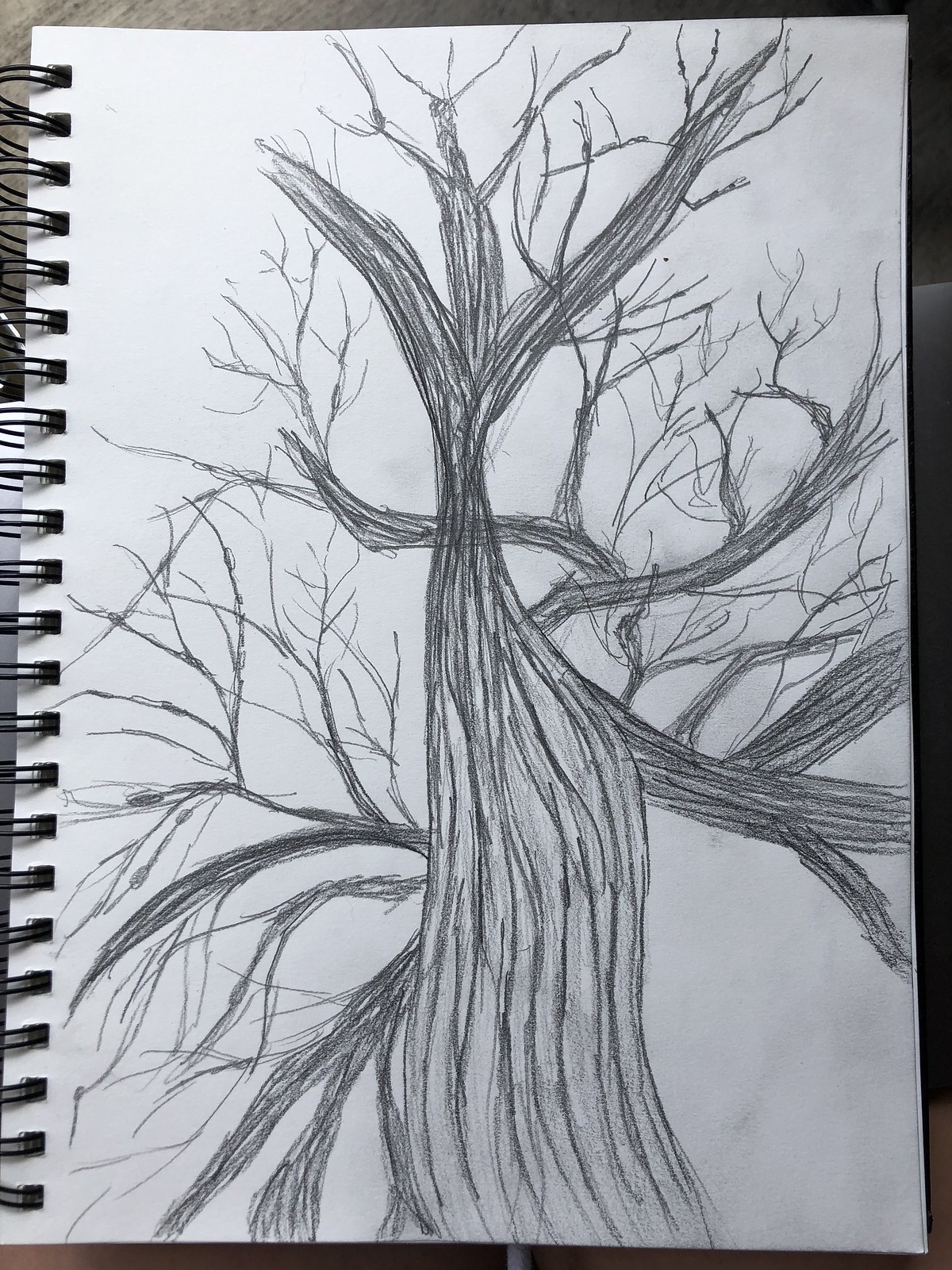This pencil drawing depicts a haunting and eerie tree, meticulously illustrated with varying shades of graphite to convey a sense of decay. The tree's gnarled branches, devoid of leaves, twist and stretch outwards from the trunk’s upper sections, enhancing its spooky appearance. The bark, textured with curved lines that flow upward and split into three distinct sections, adds to the tree’s unsettling demeanor. The background features gradations of shading, skillfully capturing the illusion of light originating from the top left corner. This light contrasts with darker shaded areas, subtly emphasizing the tree's morbid and lifeless state.